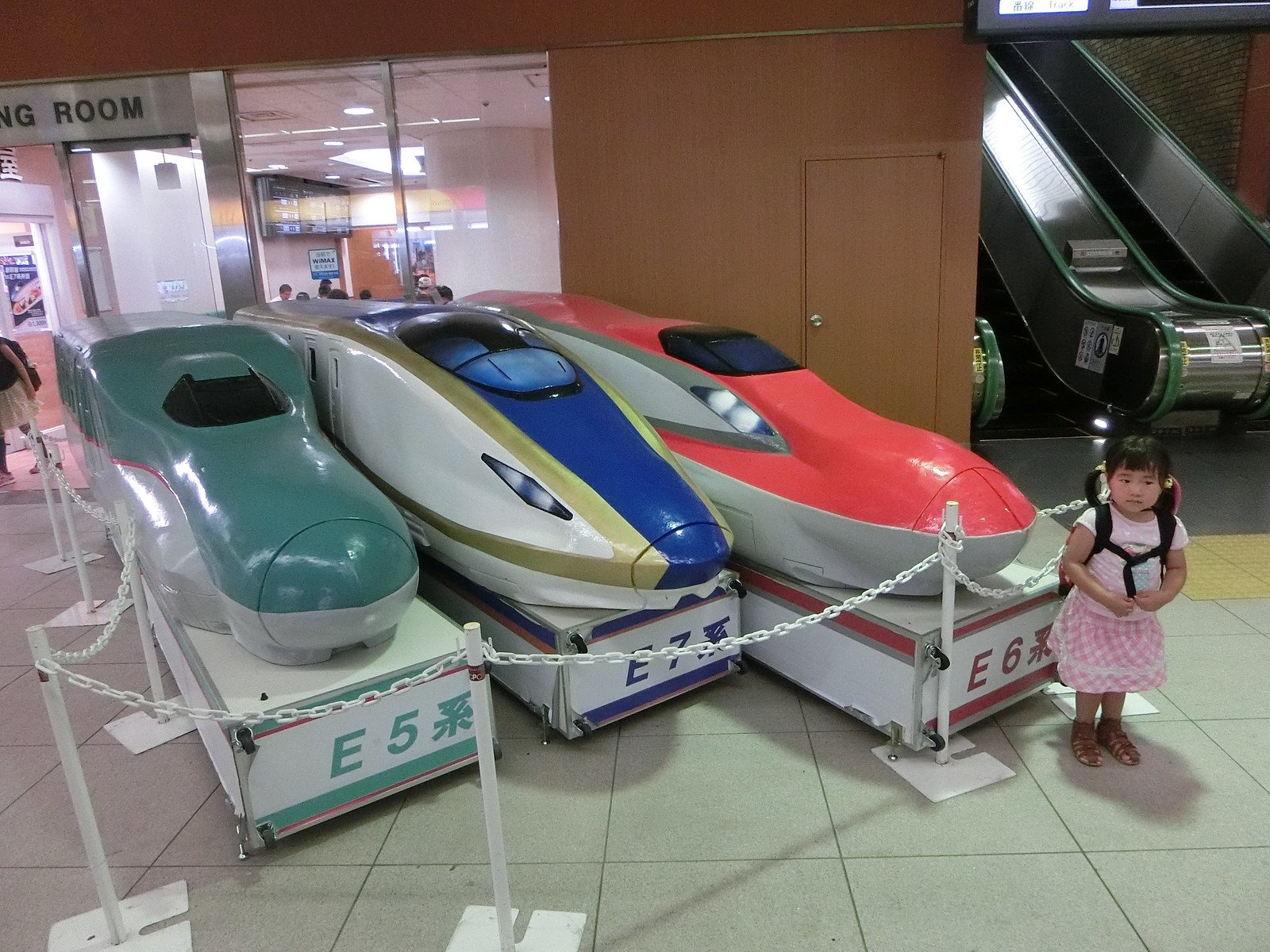This color photograph captures a bustling scene likely set in a Japanese train station or retail area, known for its characteristic blend of traditional and modern elements. Dominating the foreground are intricately crafted models of bullet trains, encased within a short white chain-link fence supported by vertical poles on square bases. Each model is detailed with Japanese characters on their bases, reading E5, E6, and E7, denoting the different train series. A small girl in a pink dress with long ponytails and a backpack stands near these models, drawing attention to the vibrant display.

The background reveals a spacious setting with white tile flooring leading to wooden paneled walls, enhancing the warm ambiance. A pair of escalators ascend toward the upper right corner, suggesting a multi-level establishment. Through the tall windows adjacent to the escalators, the heads of seated individuals are visible, possibly within a waiting room or a café. Overhead signage partially displays the word "room," indicating it could be a "waiting room." The scene impeccably captures the fusion of everyday life and the iconic culture of rail travel in Japan.